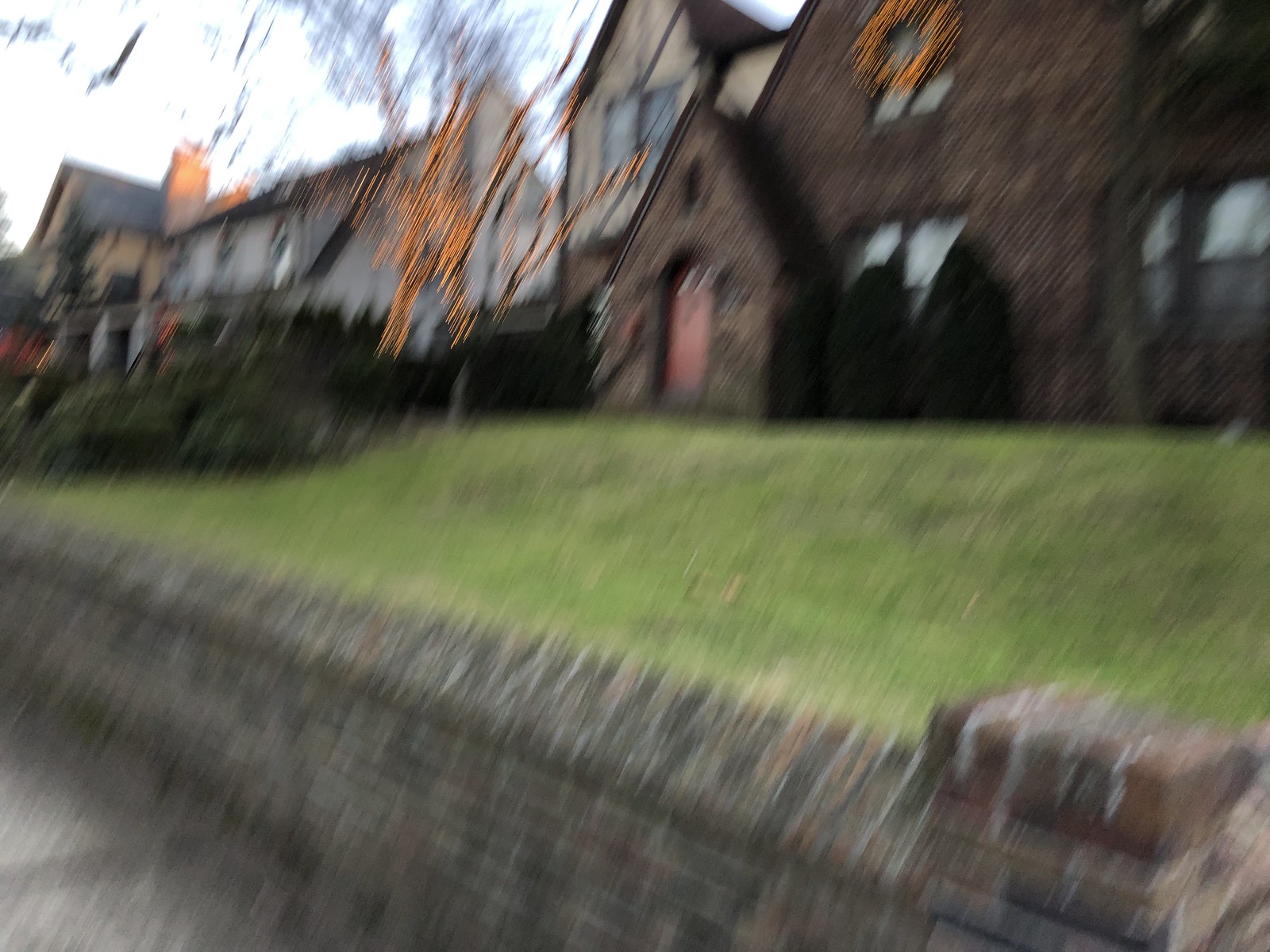A blurry photograph taken from a footpath captures a streetside scene featuring houses bathed in the muted light of a grey evening. The footpath, composed of concrete, enters the image from the bottom left corner and runs diagonally across the frame. Adjacent to the footpath is a small brick wall built from variously colored rectangular bricks in shades of brown, dark grey, and light brown. This brick barrier functions as a retaining wall, supporting a slightly elevated lawn behind it.

In the background, towards the right side of the image, stands a traditional brick house with distinct architectural features. The house boasts pointed, triangular roofs and a red wooden front door with an elegant semi-circular top. Above the door, round windows can be seen, reflecting the dull grey hues of the evening sky, adding a somber yet charming atmosphere to the scene.